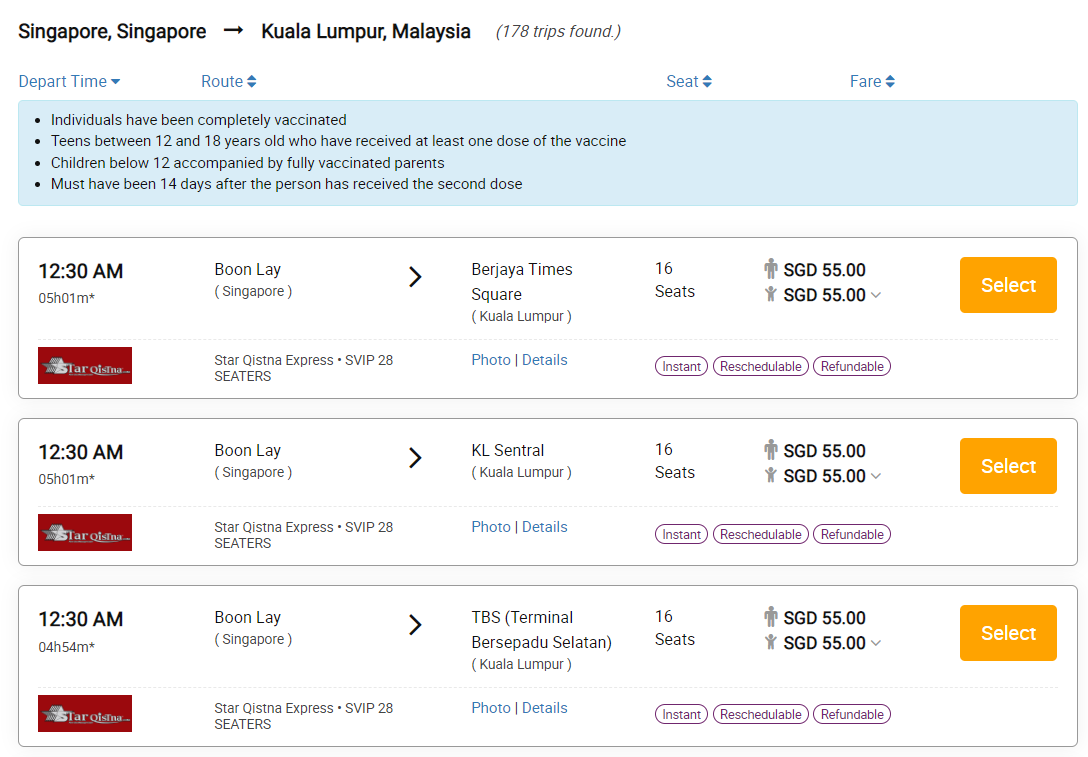This image appears to be a screenshot from a flight booking application, displaying available trips from Singapore to Kuala Lumpur, Malaysia. The header at the top shows "Singapore, Singapore" with an arrow pointing to "Kuala Lumpur, Malaysia," and a note indicating that 178 trips have been found.

Directly below the header, there are interactive options to select departure time, route, seat, and fare, each featuring dropdown menus and arrows for adjustments. Highlighted in blue is a significant section detailing the travel requirements under COVID-19 guidelines. It states that fully vaccinated individuals, teens aged 12-18 with at least one vaccine dose, and children under 12 accompanied by fully vaccinated parents can travel, provided it has been 14 days since the second dose of any eligible vaccine.

The image details three specific flights:

1. **Flight 1:**
   - **Departure Time:** 12:30 a.m.
   - **Duration:** 9 hours and 1 minute
   - **Route:** From BOON LAY, Singapore to BERJAYA Times Square, Kuala Lumpur
   - **Seats Available:** 16
   - **Price:** 55 Singaporean dollars
   - **Additional Details:** Identified as "Star Qvistna Express SVIP 28", with an external link for photos and more information. It is mentioned to be instantly reschedulable and refundable.

2. **Flight 2:**
   - **Departure Time:** 12:30 a.m.
   - **Duration:** 5 hours and 1 minute
   - **Route:** From BOON LAY, Singapore to KL SENTRAL, Kuala Lumpur
   - **Seats Available:** 16
   - **Price:** 55 Singaporean dollars
   - **Additional Details:** The flight also offers options for instant rescheduling and refunds.

3. **Flight 3:**
   - **Departure Time:** 12:30 a.m.
   - **Duration:** 4 hours and 54 minutes
   - **Route:** From BOON LAY, Singapore to TBS Terminal Bersepadu Selatan, Kuala Lumpur
   - **Seats Available:** 16
   - **Price:** 55 Singaporean dollars
   - **Additional Details:** The same conditions as the first two flights, i.e., instant rescheduling and refund options.

Each flight listing includes a prominent orange button labeled "Select." There is fine print below each option, providing details regarding the service and terms of the tickets.